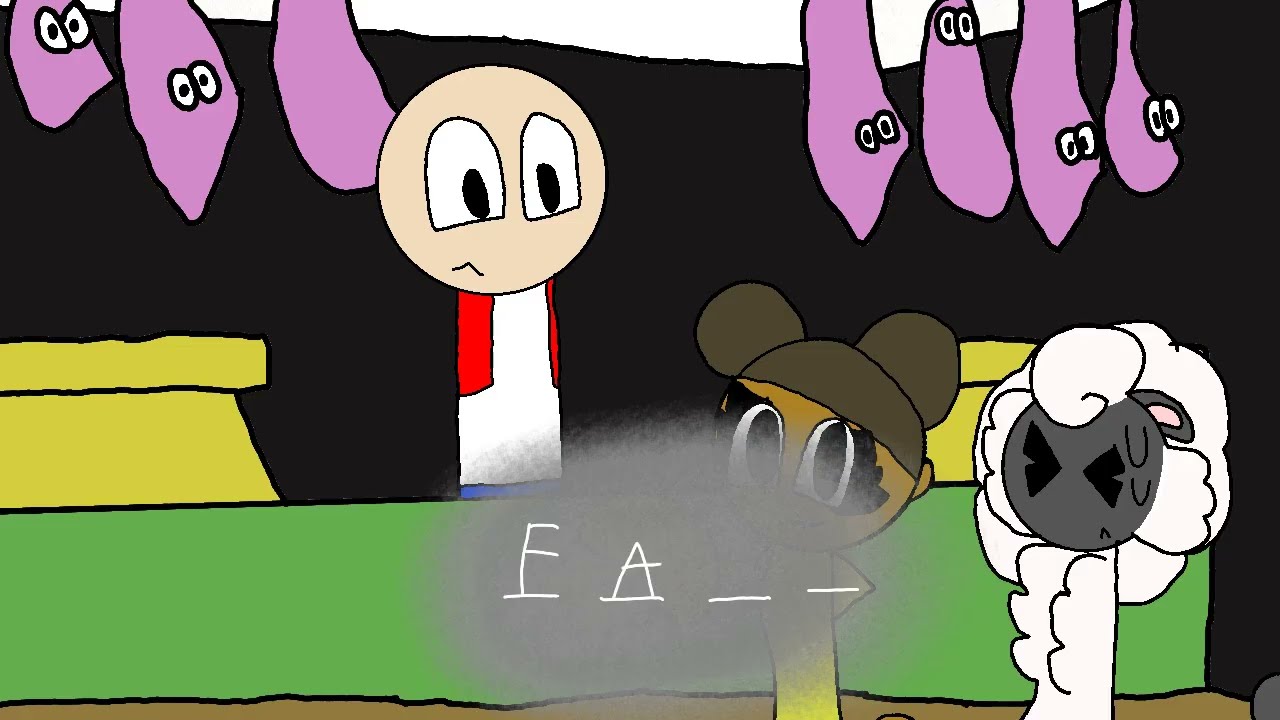This image is a hand-drawn, cartoon-style depiction from the "Amanda the Adventurer Story" game. Set against a black background, the scene features several characters and objects in various colors including purple, black, white, tan, red, yellow, green, brown, and gray.

In the foreground at the bottom right, there's a white sheep with a gray face standing next to a girl wearing a cap adorned with Mickey Mouse-like ears. Close to the center, there is a man with a round head, large eyes, and a smirk, wearing a white shirt with red sleeves and blue pants, situated behind a green counter or stage.

Suspended from the top of the image are various purple items with cartoonish eyes, resembling figures hanging in a butcher shop. To the left of the man behind the desk is a green item that looks like a scale or a box.

At the bottom of the image, there are four horizontal lines intended for a fill-in-the-blank puzzle. The first two lines are filled with the letters "F" and "A", while the remaining two are left blank. The overall style of the illustration appears to be a poorly drawn cartoon, with a mix of quirky, exaggerated features and vibrant colors.